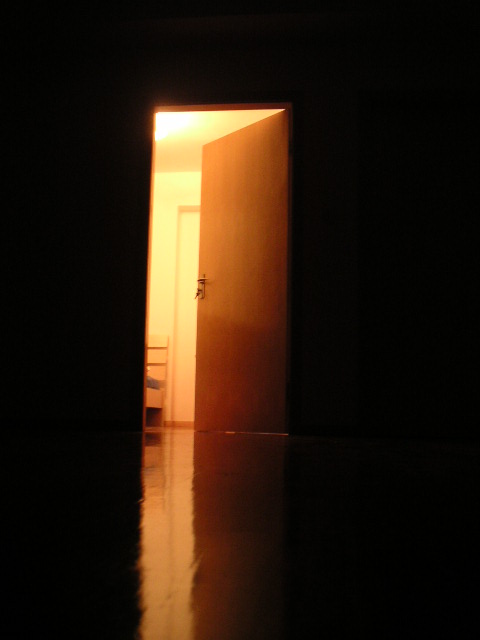This photograph captures the eerie contrast between a completely dark room and an adjacent room bathed in light. In the image, the focal point is a brown wooden door that is slightly ajar, creating a dramatic visual entry. The door's opening reveals a well-lit room where a portion of a furniture piece, possibly a chair or a bench, is visible. A light situated in the top left corner of this illuminated room highlights the surroundings. The light spills through the doorway, reflecting off the dark room's floor, enhancing the sense of depth and contrast. Within the illuminated room, there is also another door that remains closed. The image’s dark border intensifies the brightness emanating from the ajar door, making the interplay of light and shadow particularly striking.